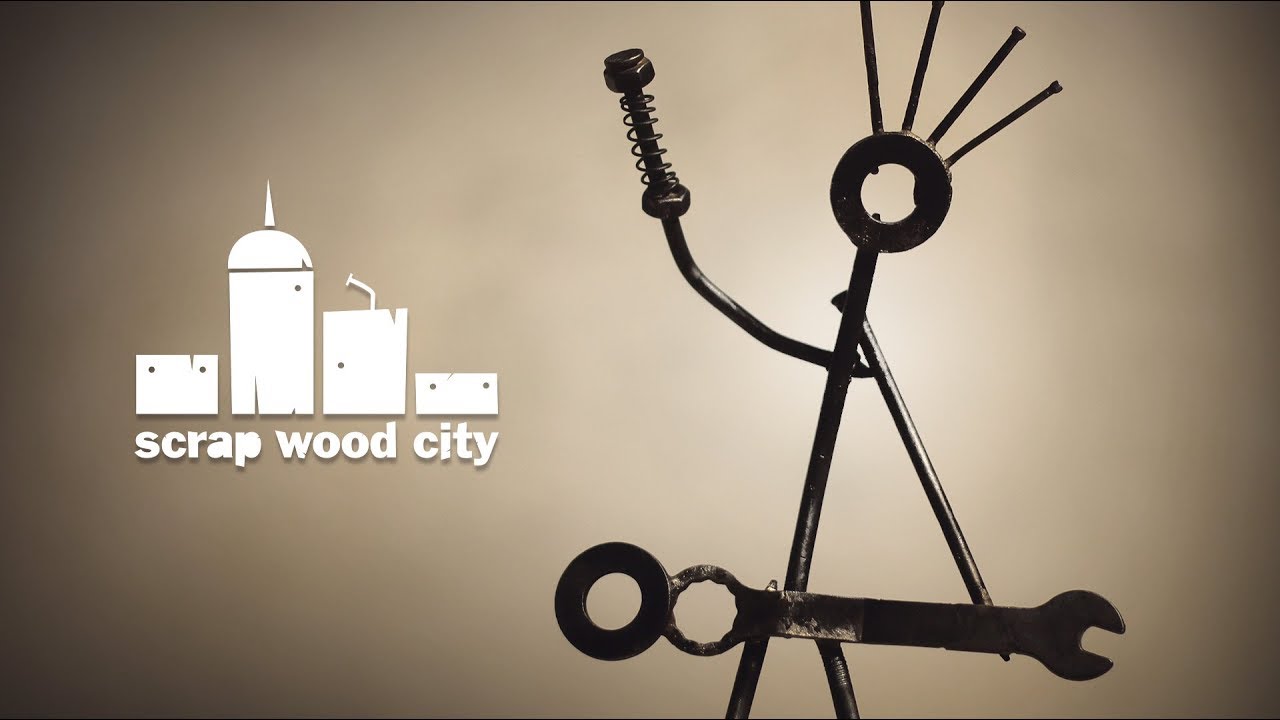The image is a striking photograph of a creative scrap sculpture set against a background that transitions from a light gray in the center to a deeper mauve in the corners, giving it a shadowy, vignetted effect. This compelling artwork features a stick figure made from various metallic components, resembling a person playing guitar. The figure's body is constructed from a nail, with two nails forming its legs. A wrench serves as the guitar, held in place with another nail, while a bent wire shapes the guitarist's right arm, holding a pen spring as if ready to strum. The figure's head is a washer adorned with three smaller nails protruding as hair, enhancing its whimsical, mechanical appearance. On the left side of the image, a bit over halfway down, is the label "Scrap Wood City," written in lowercase letters. Directly above this text is a logo depicting four wooden buildings of varying heights, some crowned with metal pieces and nails, emphasizing the theme of repurposed materials.